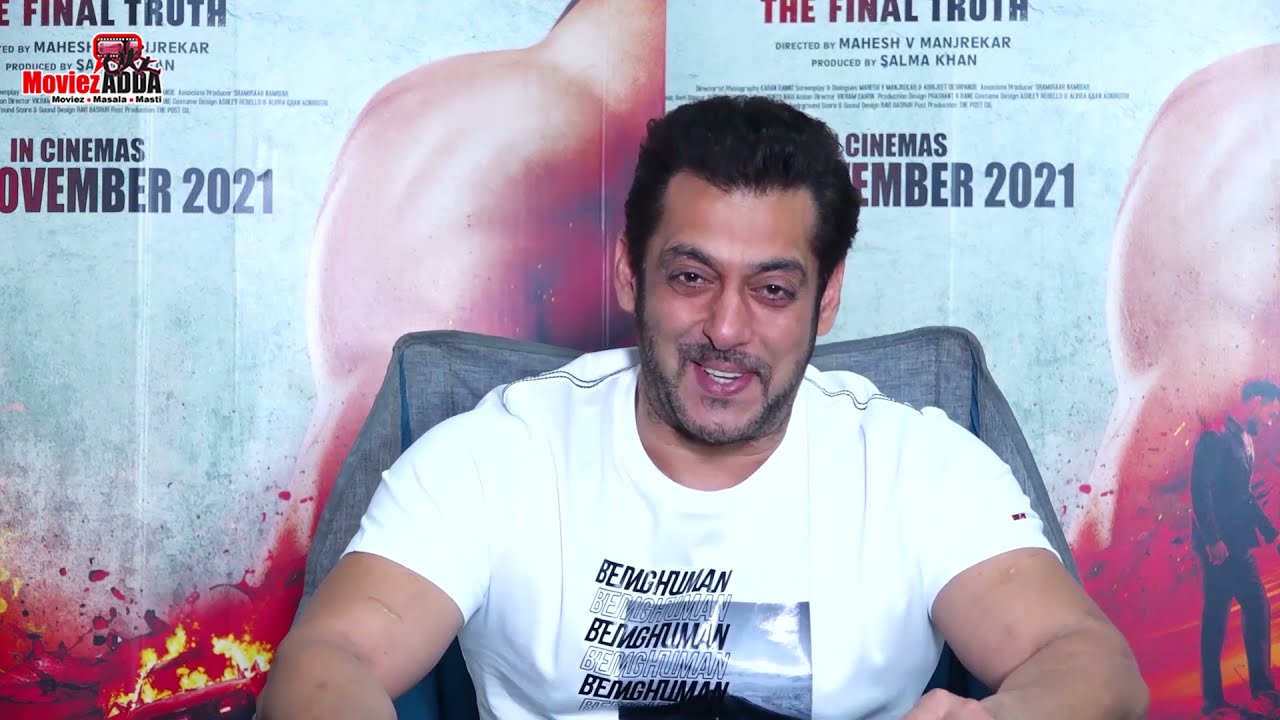In this wide rectangular image, a man of likely Indian descent sits prominently in front of a backdrop displaying movie posters. The posters, which feature light blue backgrounds and a striking design of red and yellow flames at the bottom, are mirrored on the left and right halves of the photo. At the bottom right corner of these posters, a man in a suit is visible, contributing to the intricate visual layout. The posters prominently advertise the movie "The Final Truth," directed by Mahesh B. Mandrikar and produced by Salma Khan, with a noted release in theaters set for November 2021.

The central figure is a man with light brown skin, dark brown hair, and distinctive facial features including a mustache and beard. Dressed in a white T-shirt emblazoned with the repeating words "Being Human," he sits on a gray and blue chair, smiling warmly with crinkled eyes and displaying his upper teeth. His T-shirt reveals his muscular arms, which show signs of past scarring and healed wounds. The image appears to depict an interview or media interaction, possibly sourced from the website Moviesadda, rendered in red and black font. This setting suggests that the man could be an actor, director, or a significant figure involved in the making of the highlighted film.